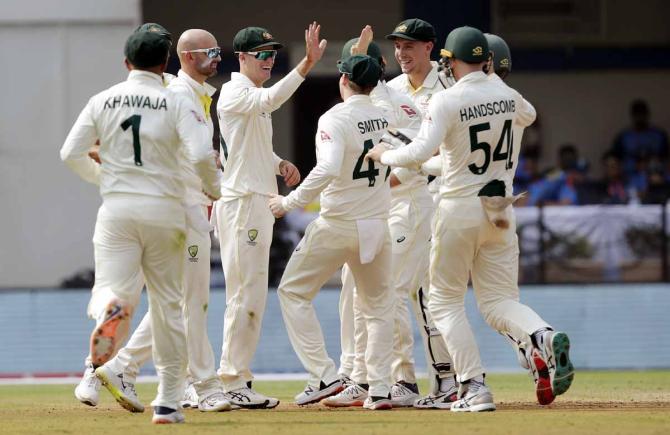The photograph captures a jubilant moment featuring a cricket team in white uniforms celebrating their victory on a verdant field enclosed by a pale blue border. The players are seen high-fiving, smiling, and laughing, and the scene is filled with a sense of camaraderie and triumph. 

On the left of the image is Kavadra, wearing number one on his back, clad in a white uniform with a cap. To his right stands a bald player sporting sunglasses, his face turned to the right. Next is Smith, number 47, also wearing sunglasses and a cap, high-fiving another teammate. The team members are diverse in their headgear; some wear helmets, others caps, while a few are bareheaded. Additionally, some players wear sunglasses, adding to the casual yet focused atmosphere.

Further to the right is Hans Gomb, number 54, who appears to be running with his name and number visible on his uniform. The celebratory mood is set against a backdrop of a blurred audience seated in the stands, capturing the essence of a lively cricket match in what seems to be a stylus port stadium.

The white uniforms of the players are distinct, with numbers and perhaps a coat of arms or crest on the right leg, and dark caps featuring gold markings. The gleaming green grass of the field contrasts with the pale blue boundary, making the momentous occasion stand out vividly.